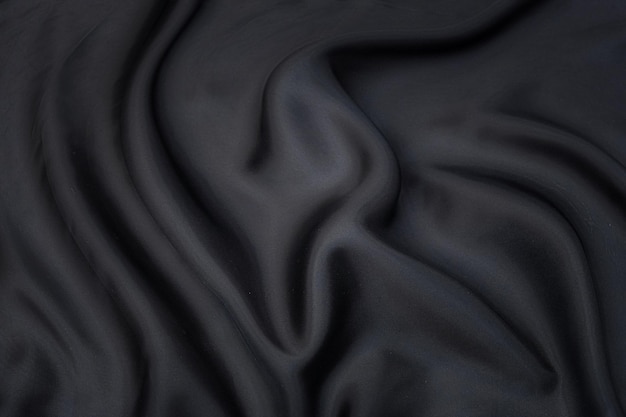The image portrays a blurry, black fabric with a silky texture, abundant folds, and a somewhat eerie appearance. On the left side, the folds curve from the top down to the bottom, while in the middle part of the fabric, a shape akin to a human ear is noticeable. The right part of the fabric features folds that curve horizontally from the center to the edge. The overall effect is ghostly, with the drapery's wavy, uneven lines and dark divots creating a haunting visual. In the center, there appears to be a faint, ghostly white circle, adding to the spectral ambiance of the image.